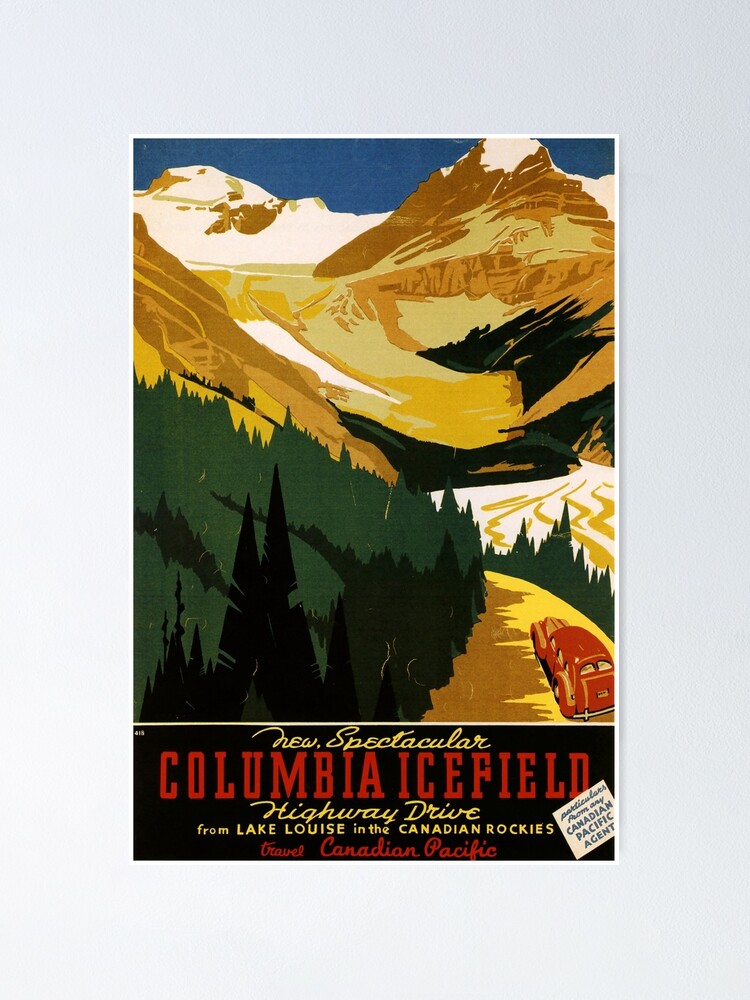This retro-style travel advertisement, likely dating back to the 1940s or 1950s, features an illustrated depiction of the Canadian Rockies beneath a deep blue sky. The mountains are rendered in various shades of brown with white snowcaps at their peaks. A winding yellow road cuts through the bottom right of the Rockies, flanked by lush evergreen trees. A red car is seen driving along this scenic route. Below this captivating scene, the poster has a black rectangle with text in varying colors: "New Spectacular" in beige-yellow, "Columbia Icefield" in red, and "Highway Drive from Lake Louise in the Canadian Rockies" also in beige-yellow. The tagline "Travel Canadian Pacific" appears underneath. The poster also includes a white square in the lower right corner, containing some blue text related to contacting a Canadian Pacific Agent. The entire image is framed with a thick, light blue border, enhancing its vintage charm.